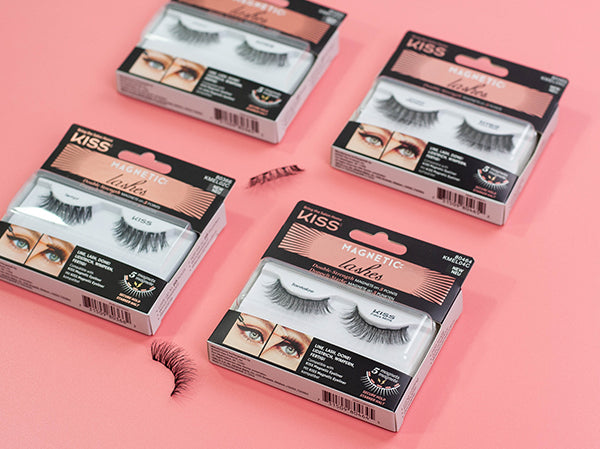This image is set against a pink background and features four packages of Kiss brand magnetic false eyelashes, along with two additional sample eyelashes resting directly on the surface. The packages are arranged in a grid-like pattern, with two on top and two below, slightly angled to the left. Each package is black with a transparent window that displays two incredibly long and lush, albeit slightly spidery, eyelashes. The top left corner of each package is branded with "Kiss," and the text "Magnetic Lashes" is prominently displayed toward the top center. The lower section of each package features instructional illustrations on how to apply the lashes, accompanied by photos of eyes wearing the lashes. The packaging also includes some pink decorative elements and a barcode. The overall presentation highlights the product's premium and eye-catching design.